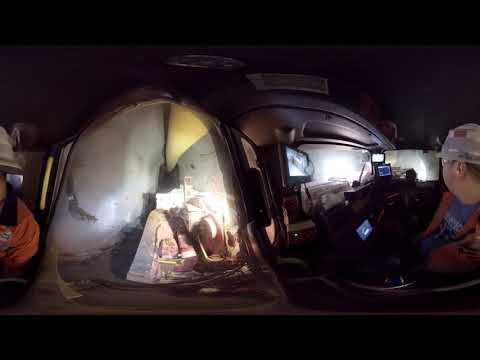In the photo, a construction or industrial worker, positioned towards the right side, sits in front of illuminated computer screens. The worker is attired in an orange vest, blue shirt, and a white safety helmet. The scene appears to depict the inside of a vehicle or industrial environment. The background is predominately dark, with black bars running horizontally across the top and bottom of the image. To the left, partially visible, is another worker, identifiable by the shoulder of their orange vest. The middle left side features a lit area with gray walls and yellow objects, possibly industrial equipment.